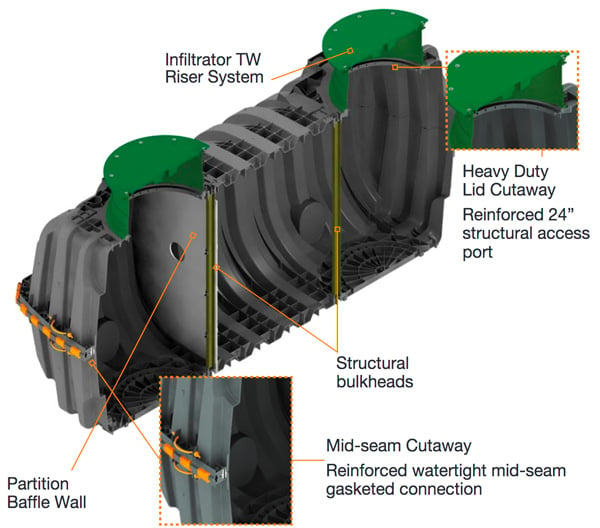The image presents a detailed cutaway drawing of a gray industrial component, possibly related to water systems or automobile engineering. The main body of the unit is a dark battleship gray, segmented with bright orange pieces that securely hold the structure together. Intricate green parts, labeled as "Infiltrator Riser Systems," are integrated into the assembly. Notable labeled elements include a "Partition Baffle Wall" with a distinct hole, and a "Structural Bulkhead." An inset image highlights a "Mid-Seam Cutaway Reinforced Watertight Mid-Seam Gasketed Connection," emphasizing the unit's waterproof characteristics. Additional labeling specifies a "Heavy Duty Lid Cutaway Reinforced 24-inch Structural Access," contributing to the overall robustness and functionality of the component. The descriptive annotations and cutaway views provide a comprehensive insight into the internal construction and key features of the system.